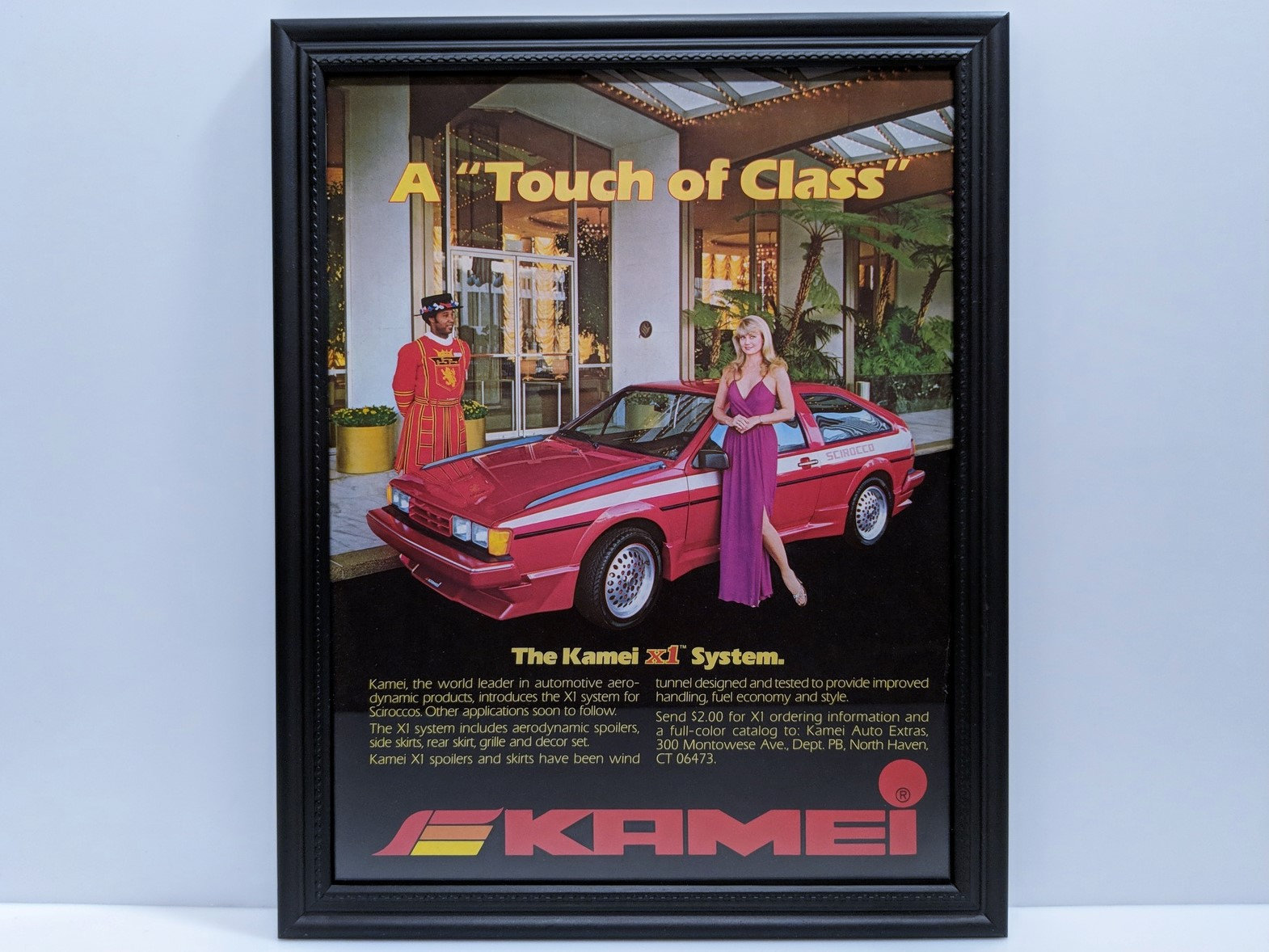This advertisement poster, set in a black braided frame against a light blue wall, features a vintage scene that evokes the 1980s. At its center is a small, sporty, red two-door car with a distinctive white stripe along its side and two blue stripes edging the hood. In front of the driver's door stands an elegant blonde woman in a strapless, purple evening gown with a high slit, revealing her high heels. Just behind the front of the car, a man dressed as a hotel bellhop in a red uniform with gold insignia and a black hat is present, enhancing the scene's opulence. The top of the poster boldly states "A Touch of Class" in yellow text, capturing the theme of sophistication. Below the car is the text "The Kamei X1 System," followed by a detailed description of Kamei's aerodynamic products, featuring spoilers, side skirts, rear skirts, grills, and decor sets, all designed to improve handling, fuel economy, and style. The advertisement concludes with a call to action, inviting viewers to send $2 for a full-color catalog from Kamei Auto Extras in North Haven, Connecticut. The brand name "Kamei" is prominently displayed in red letters with a large circle dotting the 'I', ensuring brand recognition.